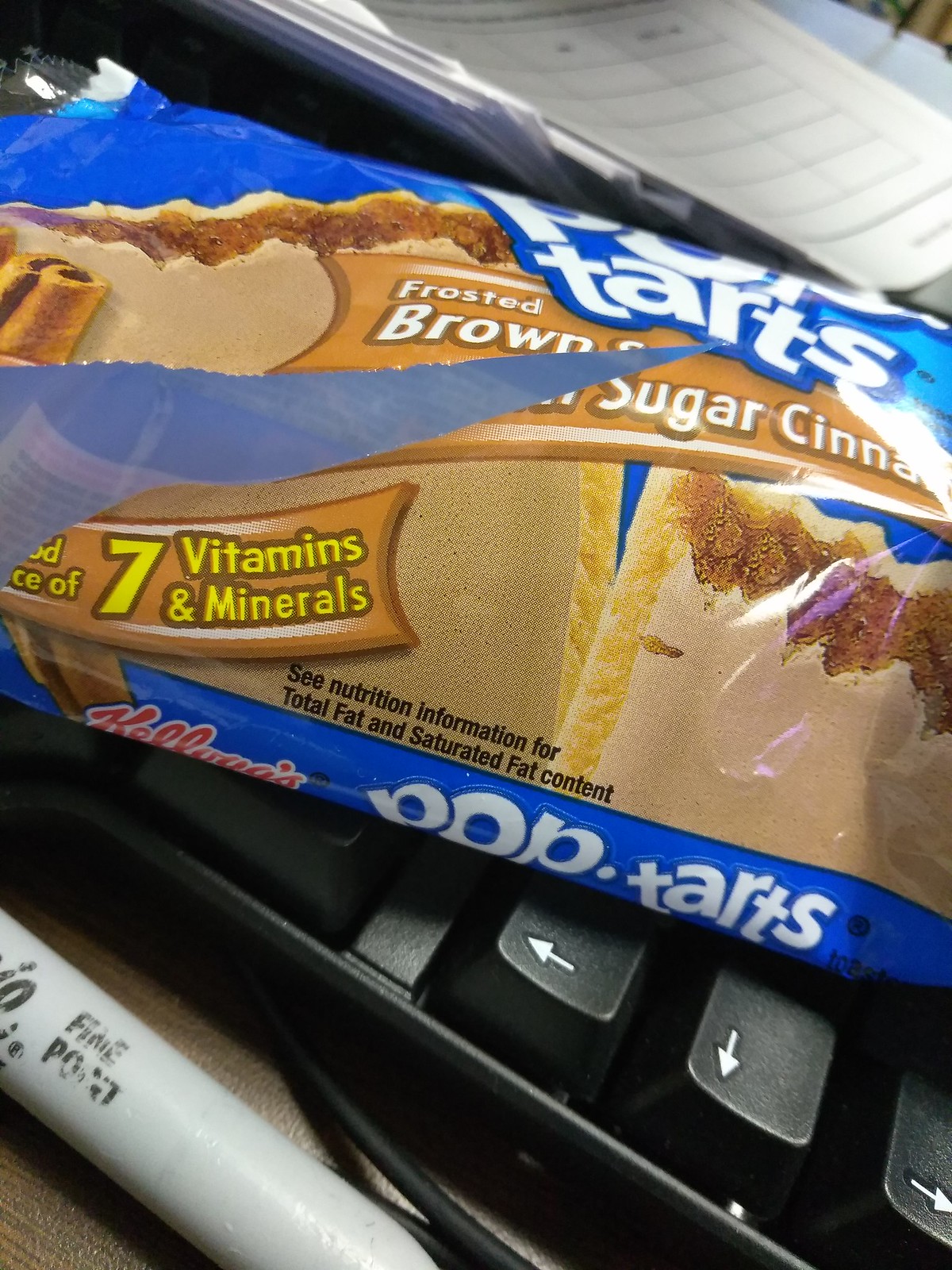This image depicts a close-up of a torn-open blue Pop-Tarts wrapper, specifically for the Frosted Brown Sugar Cinnamon variety, showcasing the Kellogg's Pop-Tarts branding prominently in white letters. The wrapper features large images of the Pop-Tarts broken in half, revealing the brown sugar cinnamon filling inside. The package touts "seven vitamins and minerals" and "Kellogg's" in yellow writing. The ripped-open wrapper, now void of Pop-Tarts, rests on a black keyboard with white annotations, which is placed on a brown wooden desk. In front of the keyboard lies a fine-point Sharpie marker, with some papers and a few blue tabs visible behind the keyboard, adding to the cluttered office desk setting.